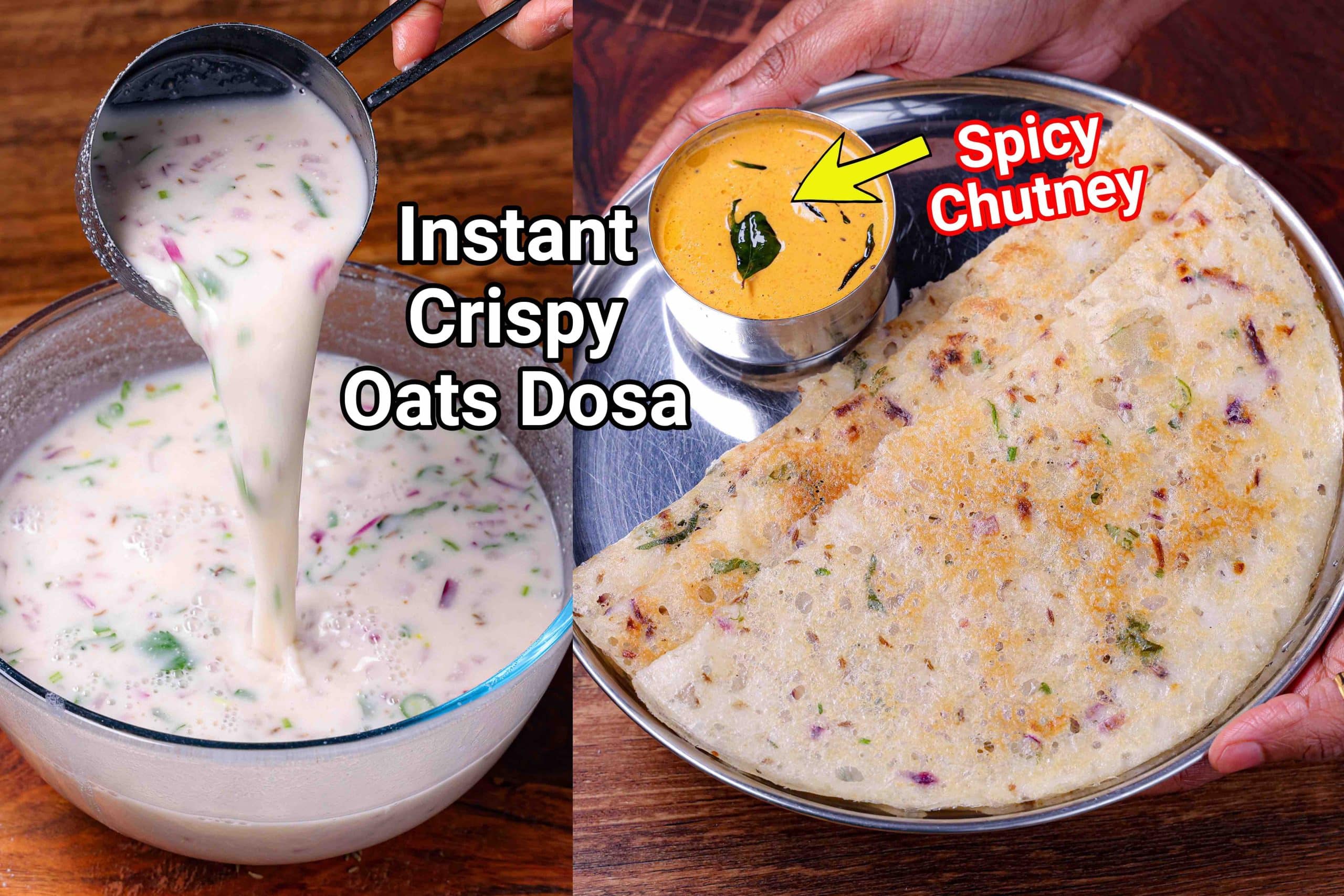The advertisement for Instant Crispy Oats Dosa captures two vibrant and detailed color photographs showcasing the preparation and presentation of the dish. In the left image, a hand pours a ladle of a white, speckled mixture containing red and green pieces into a glass bowl, presumably illustrating the process of making the dosa batter. The right image features two hands holding a round silver tray that displays two folded and crisp dosas, resembling a blend between crepes and quesadillas. Also on the tray is a small silver dish labeled "Spicy Chutney," containing a vivid orange sauce speckled with green chili peppers and garnished with a leaf. The dosas are colorful, with visible red, green, and purple specks, emphasizing the ingredients used. The bright and focused images beautifully highlight the textures and colors of the food, making the dish appear both appetizing and visually appealing.